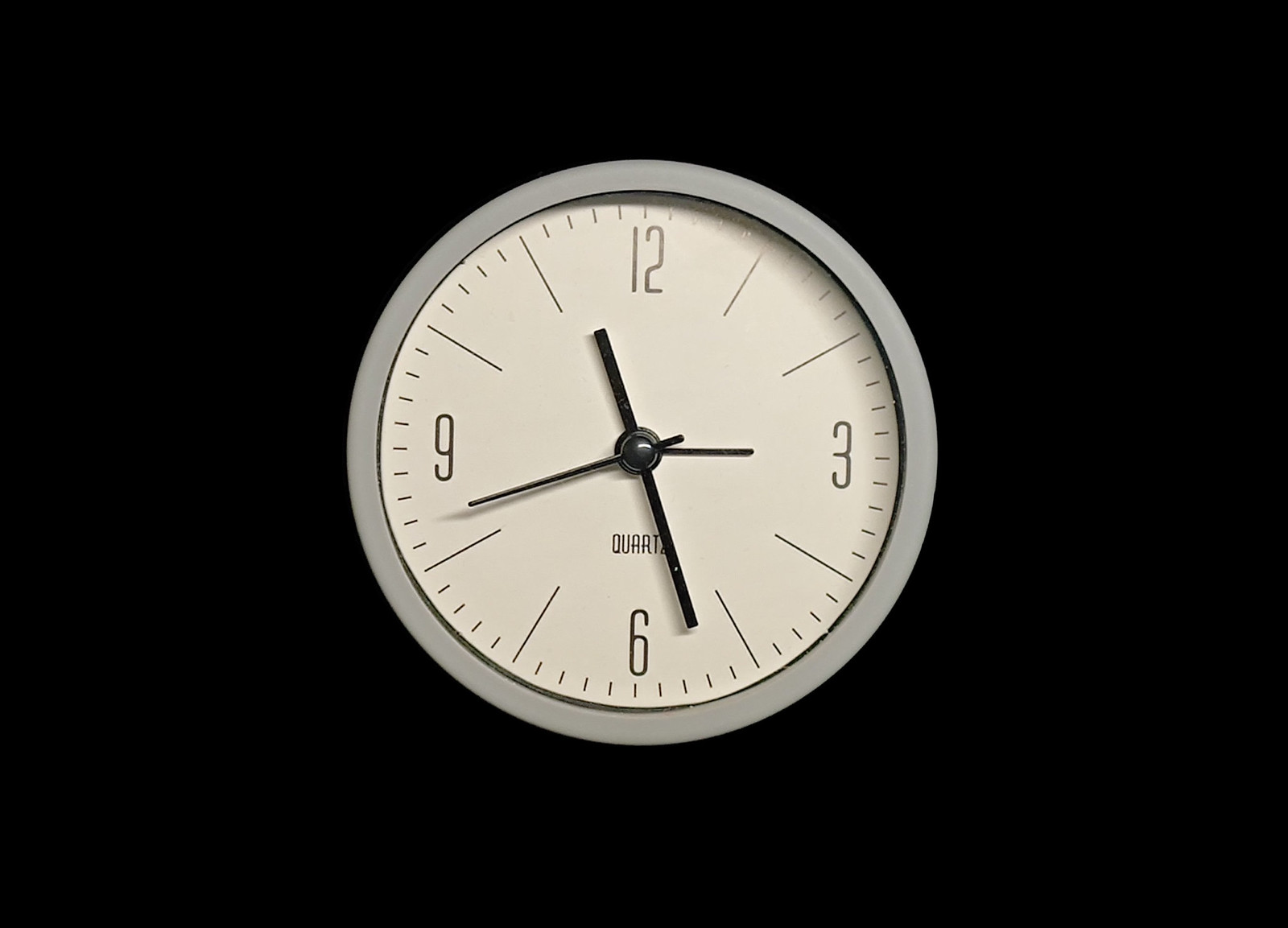This is a photo of a round wall clock featuring a sleek silver trim on its exterior. The clock face displays only the numerals 12, 3, 6, and 9, with dashes marking the intervals in between. Positioned near the 6 o'clock mark is the word "quartz." The clock is equipped with three black hands – minute, hour, and second – all contrasting against a black inner rim. The backdrop behind the clock is a solid black, enhancing its modern and minimalistic design. The image appears to be computer-generated, adding to its polished and refined aesthetic.